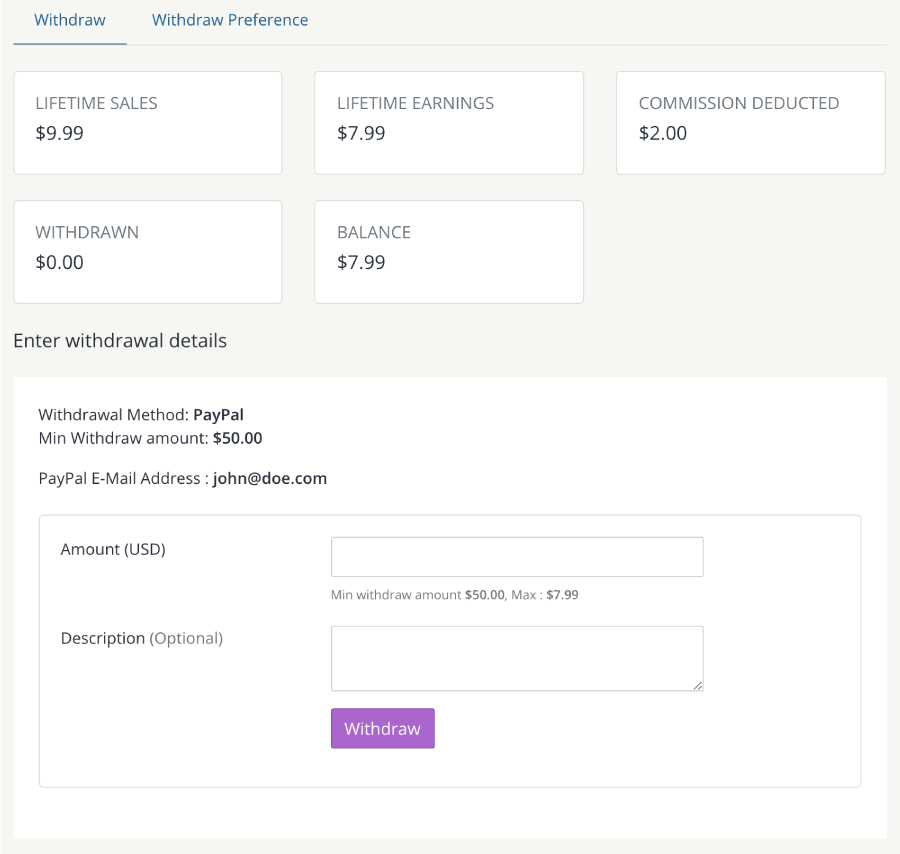The image is a vertically oriented rectangle with a cream-colored background. At the very top, there is text written in black and blue. The blue text, which is underlined, reads "Withdraw," and to its right, it says "Withdraw Preference" in black.

A thin gray line separates this top section from the next.

Below this line are five white boxes outlined in gray:
- The first box at the top left displays "Lifetime Sales: $9.99."
- The box to the right of it reads "Lifetime Earnings: $7.99."
- The third box at the far right shows "Commission Deducted: $2."

On the row below:
- The first box on the left says "Withdrawn: $0."
- The box next to it reads "Balance: $7.99."

Further down the page, there is a section titled "Enter Withdrawal Details."

In this section, a larger white box contains the following text in black:
- "Withdrawal Method: PayPal"
- "Minimum Withdrawal Amount: $50"
- "PayPal Email Address: johnatdoe.com"

There is an individual box outlined in gray within this larger section. Inside it, there are two smaller, blank fields labeled "Amount USD" and "Description."

At the bottom of the image, there's a purple box with white text that reads "Withdraw."